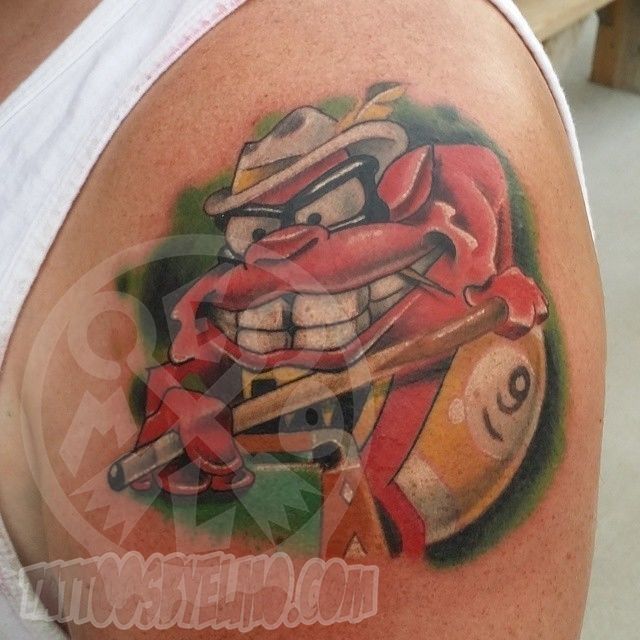This image showcases a detailed tattoo on a man's shoulder, illuminated against a grey, indistinct background. The man is wearing a sleeveless white vest, displaying a red, cartoonish demon-like creature with steely black eyes and prominent white teeth. The creature is depicted playing pool, holding a pool cue. It wears black-framed glasses and a white fedora hat adorned with a yellow headband and feather. Next to the creature is a white billiard ball with a yellow stripe, marked with the number nine. The green background of the tattoo enhances the vivid details of the demon character. Below the tattoo, a watermark is visible, reading "tattoosbylime.com."